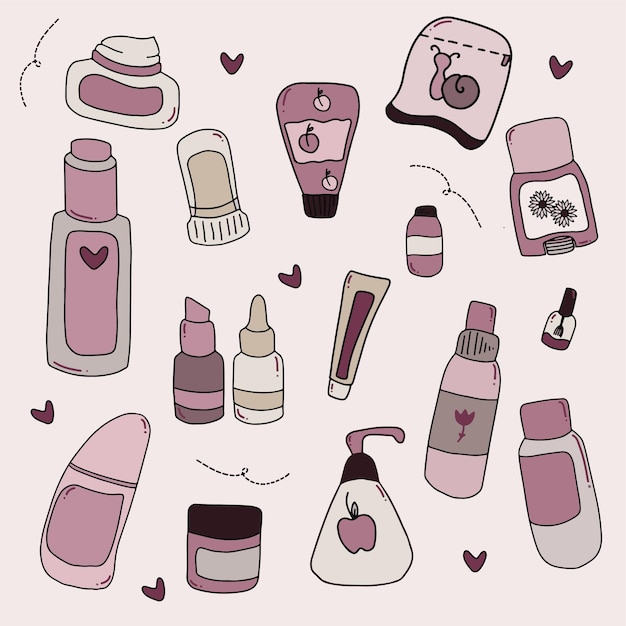This image features a cartoonish and kid-friendly assortment of beauty and makeup products, set against a pale pinkish-cream background. The whimsical design includes a variety of cosmetics such as lipstick, bottles of lotion, deodorant, nail polish, face creams, moisturizer, cuticle oil, and perfume. These items are presented in a soothing color palette of pinks, purples, khakis, tans, and beiges. Some distinctive items include jars with open tops, a twist-tube deodorant, a tube with a pump top, and a zippered pouch adorned with a flower and a snail. Scattered throughout the image are cute, drawn hearts in shades of magenta and purple, complemented by dotted squiggly lines reminiscent of a bee's flight path. The overall aesthetic of the graphic is reminiscent of pre-designed Canva prints, aimed at appealing to younger girls with its playful and soft styling.